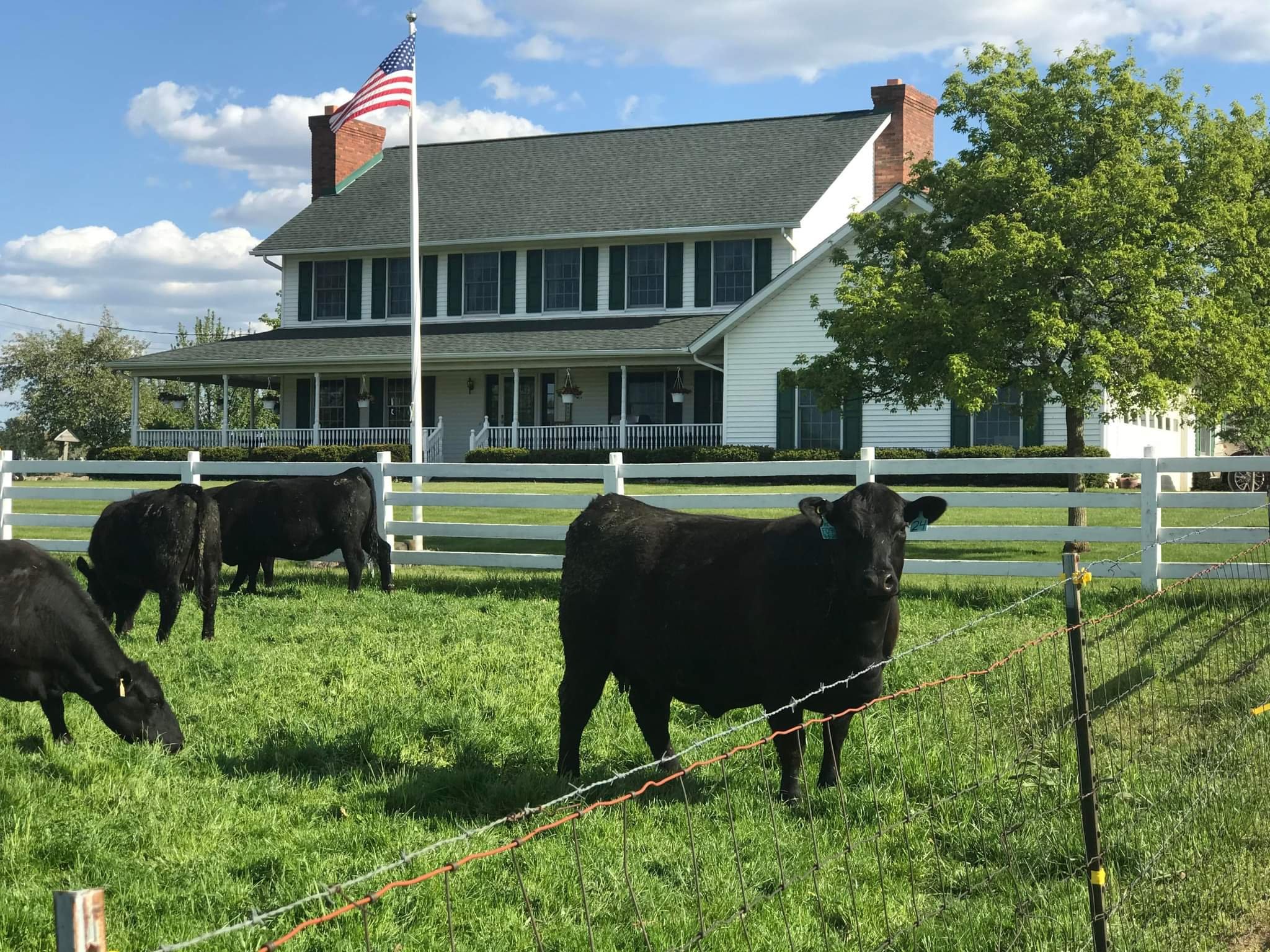In this picturesque farm scene, four black cows graze contentedly on the lush, green grass, with one cow inquisitively gazing directly at the photographer. They are bordered by a barbed wire fence in the foreground and a pristine white fence further back. Behind the cows stands a charming white farmhouse, complete with two fireplaces situated at either end. The house boasts a spacious, covered front porch that extends the full length of the structure, providing ample space for relaxation. To the right side of the house, a garage is subtly visible. Adding to the idyllic setting, a stately tree graces the front right of the house, while a flagpole stands proudly to the left.